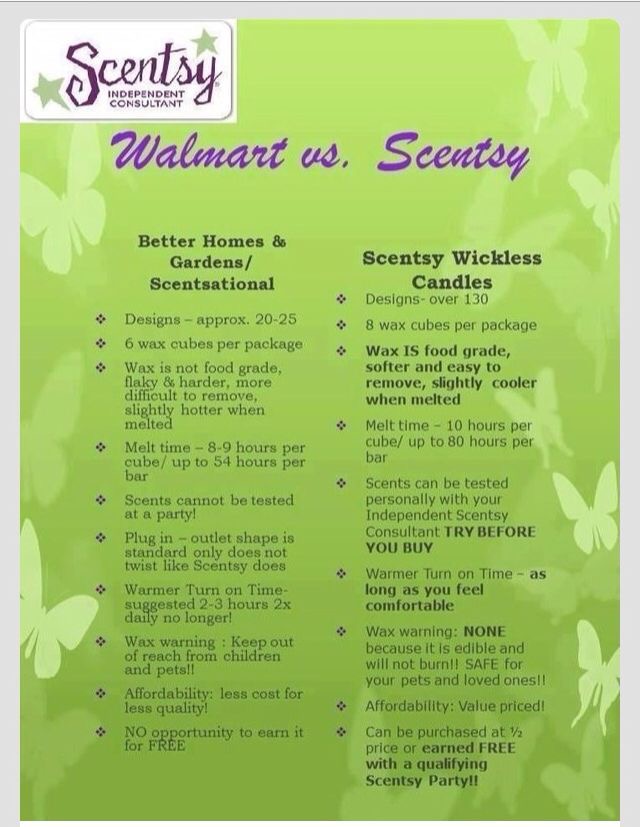The promotional flyer features a lime green background with white butterfly outlines scattered across two columns. At the top, purple text reads "Walmart vs. Scentsy." The main text is in black and compares the benefits and drawbacks of Better Homes and Gardens Sensational wax cubes to Scentsy Wickless Candles. Key details include:

- **Better Homes and Gardens Sensational:** Features 20-25 designs, each package containing 6 wax cubes. The wax is described as not food grade, flaky, harder to remove, and slightly hotter when melted, with a melt time of 8-9 hours per cube, totaling up to 54 hours per bar. The plug-in outlet shape is standard but doesn't twist like Scentsy's. The warmer should be used for 2-3 hours, twice daily. There is a warning to keep the wax out of reach from children and pets.
- **Scentsy Wickless Candles:** Compared to Walmart, it boasts over 130 designs and 8 wax cubes per package. Advertised for its ability to be purchased at half price or earned for free with a qualifying Scentsy party, where scents can also be tested.

This detailed comparison highlights key product features and usage recommendations while emphasizing Scentsy's superior variety and party perks.